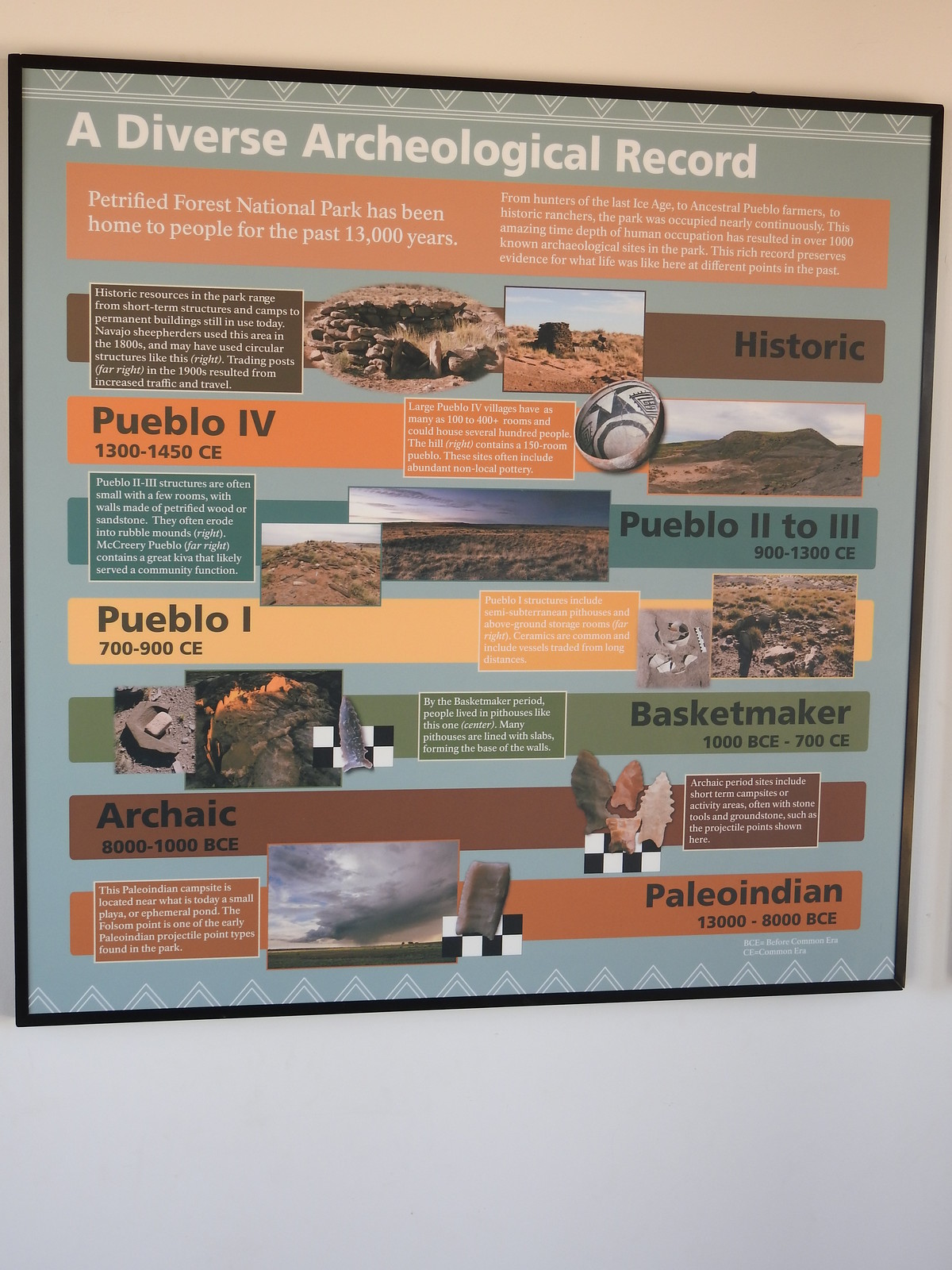The image depicts a large framed poster hanging on a wall painted in a combination of light pink and light gray. The poster features a black border and is filled with detailed information about the archaeological history of the Petrified Forest National Park. At the top of the poster, set against a bluish-green background, the headline "A Diverse Archaeological Record" is written in bold white font. 

Beneath the headline, an orange strip details the park's extensive timeline of human habitation, highlighting that the area has been occupied for over 13,000 years, from hunters of the last Ice Age to ancestral Pueblo farmers and historic ranchers. The poster underscores that this rich history has resulted in over 1,000 known archaeological sites within the park.

Immediately below this, several horizontal strips in different colors (brown, orange, green, yellow, dark green, and dark brown) categorize the archaeological record into various time periods, each featuring relevant text and images. Each strip contains boxes with descriptions and corresponding images:

- **Historic (Brown Strip):** Highlights Navajo sheep herders' circular stone structures from the 1800s and trading posts from the 1900s.
- **Pueblo 4 (Orange Strip, 1300-1450 CE):** Describes large villages with 100-4000 rooms, emphasizing non-local pottery and hill structures.
- **Pueblo 2-3 (Green Strip, 900-1300 CE):** Details small structures made of petrified wood and sandstone, including a significant kiva.
- **Pueblo 1 (Yellow Strip, 700-900 CE):** Mentions semi-subterranean peat houses, storage rooms, and traded ceramics.
- **Basketmaker (Dark Green Strip, 1000 BCE to 700 CE):** Discusses peat houses with slab-lined walls and includes images of archaeological remains.
- **Archaic (Dark Brown Strip, 8000 to 1000 BCE):** Covers short-term campsites, stone tools, and projectile points.
- **Paleo-Indian (Orange Strip, 13000 to 8000 BCE):** Depicts a campsite near a small playa, with a Folsom point and other artifacts.

Overall, the poster is a comprehensive graphical display, blending text and images to showcase the archaeological significance and continuous human occupation of the Petrified Forest National Park over thousands of years. Footnotes at the bottom clarify the abbreviations BCE (Before Common Era) and CE (Common Era).